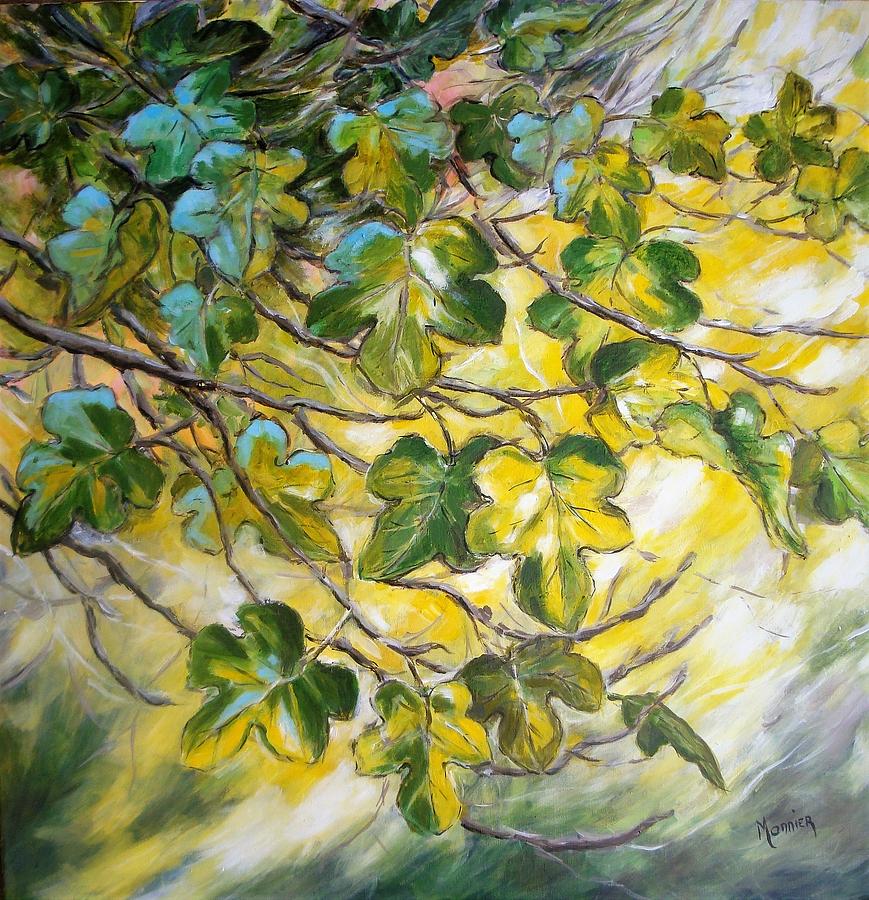This vertical rectangular painting vividly captures a cascade of green leaves with three to five lobes, arranged against a dynamic sky background. The leaves, attached to thin, dark brown branches accented with lighter hues and white highlights, weave intricately, creating a dense, intertwined network. The foliage transitions in color from dark green with blue undertones in the upper left, to more vibrant greens and yellows with white tinges towards the lower right. The background features a luminous center with a mix of yellow and white, suggesting sunlight piercing through clouds, which gradually darkens towards the edges with shades of blue, particularly in the upper left, transitioning to gray and green in the lower right. This dense arrangement of branches and leaves creates the impression of being almost impenetrable in parts, enhancing the complexity and texture of the piece. The painting, likely made with textured acrylic paint, allows one to feel the bumps and ridges of the layered strokes. In the lower right corner, the artist has signed with a subtle gray inscription reading "MANNIER." The atmospheric background, with its suggestive fog and wind-like movement, further accentuates the lively and vibrant nature of the scene, making the artwork a testament to the artist’s skill and attention to detail.